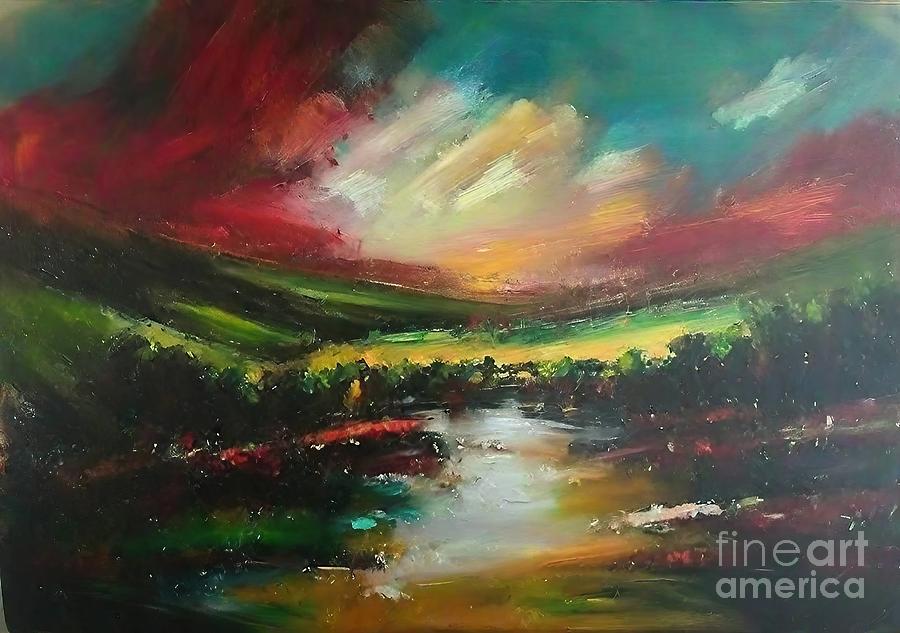This Fine Art America painting is an abstract landscape rendered with broad, expressive strokes. Dominating the top of the image are dynamic vertical streaks in red, complementing a dramatic sunset sky filled with hues of orange, yellow, and dark blue, creating an impression of an angry, turbulent atmosphere with cloudy formations. Below this fiery sky is a row of green elements sloping upwards on either side, resembling hills. The middle section is filled with rounded strokes of greens and yellows, suggesting the presence of bushes. Traversing the center of the scene from top to bottom is a stream depicted in white and yellow, flanked by dark green and red strokes, hinting at thick vegetation with some bluish-green spots perhaps resembling lily pads and intermittent white strokes that could represent logs or small animals. The painting's color palette features a harmonious blend of blue, red, yellow, and green, enhancing its abstract yet recognizable representation of a valley landscape, complete with suggestions of trees and distant farmland. In the lower right corner, the painting is marked "Fine Art America."